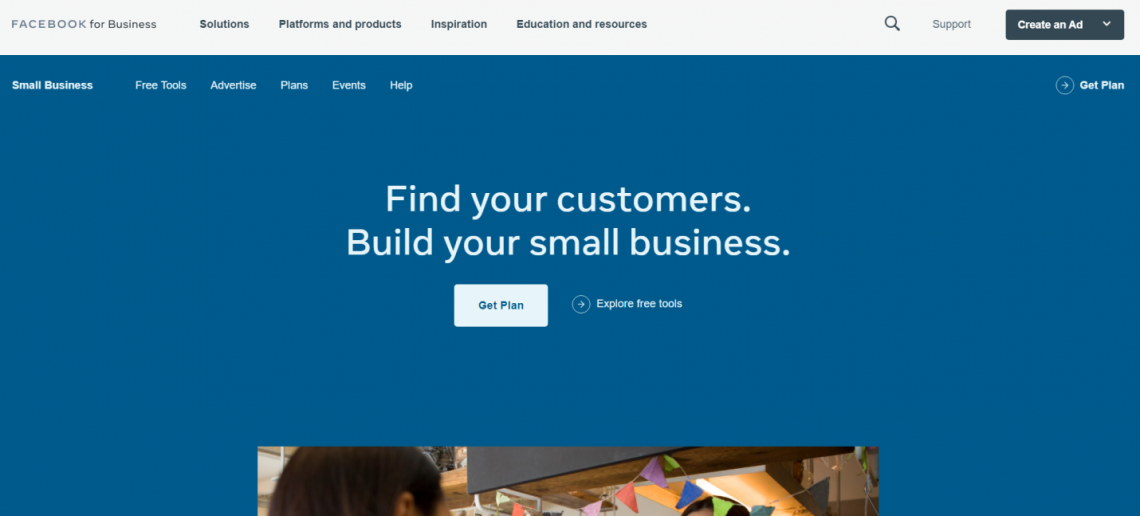The image is a rectangular banner with its longer side spanning horizontally from left to right. It features three main sections.

The top section has a light gray border with black text. This area includes the following headings: "Facebook for Business," "Solutions," "Platforms and Products," "Inspiration," and "Education and Resources." Towards the right side, there are a few icons and buttons: a search icon, a support option, and a black box with white text that reads "Create an Ad."

The middle section is predominantly blue with white text. In the top left corner of this blue section, the text reads "Small Business." Moving towards the center of this section, the text includes "Free Tools," "Advertise," "Plans," "Events," and "Help." On the far right, it says "Get Plan" in white text. In the center of this blue area, in larger font, the phrases "Find your customers." and "Build your small business." are prominently displayed. Below this text, there is a white box with blue writing that says "Get Plan," and next to it, additional text reads "Explore Free Tools."

At the bottom of the banner, an image partially appears from the bottom edge, though its content is not clearly discernible.